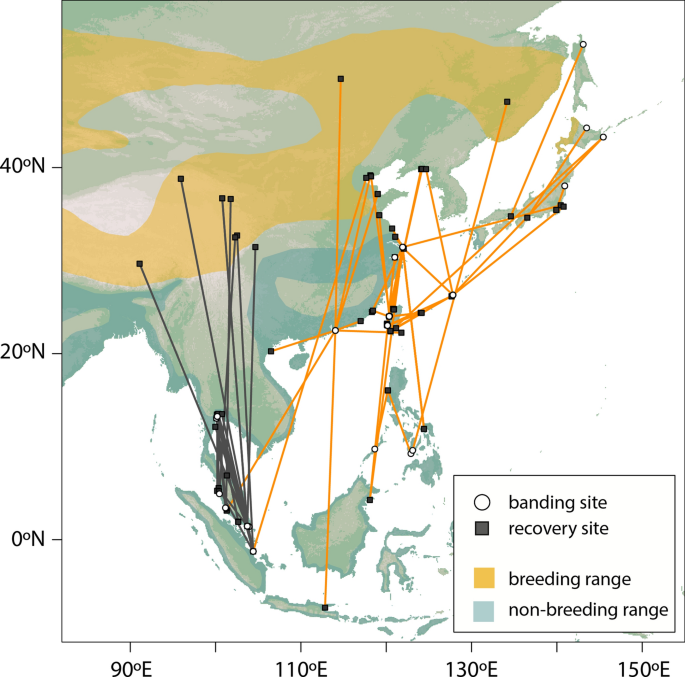The image depicts a detailed line map, likely representing a geographical area in Asia, featuring various indicators of bird activity. In the bottom right corner, there is a white rectangle serving as a legend. It describes different symbols: a white circle for banding sites, a black square for recovery sites, a yellow square for breeding range, and a green square for non-breeding range. The map is annotated with longitude lines at 90 degrees E, 110 degrees E, 130 degrees E, and 150 degrees E, and latitude lines at 0 degrees N, 20 degrees N, and 40 degrees N. Black and orange lines connect various points, indicating paths or routes relevant to the mapped activities. The primary colors on the map are white, black, yellow, and shades of green.